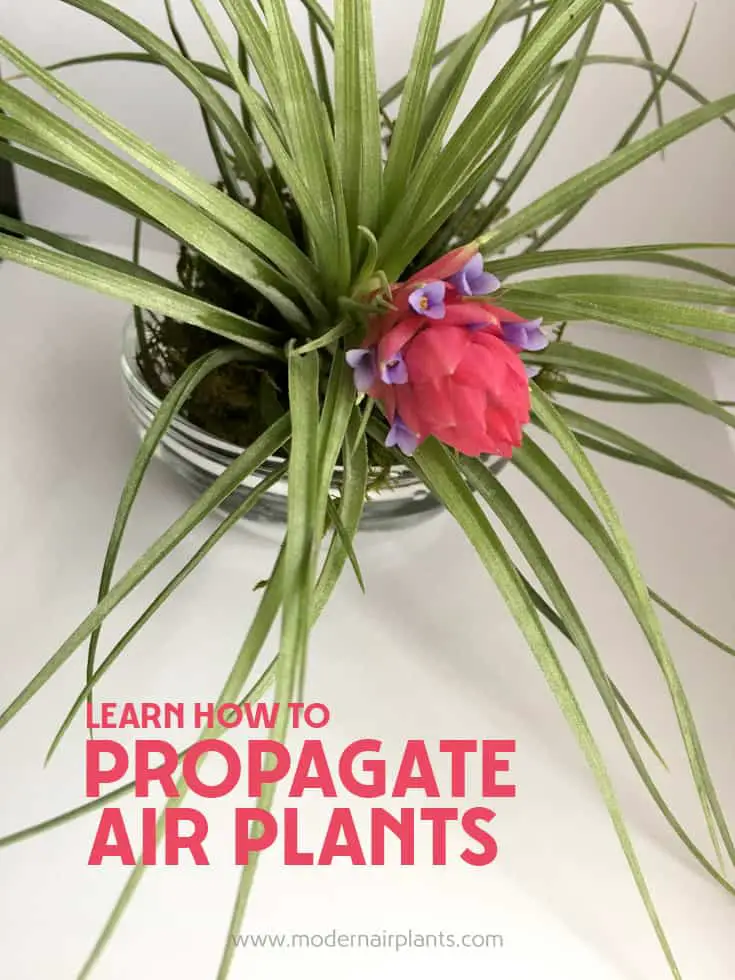The cover of the book prominently features a vibrant green spider plant housed in a shiny silver planter on a white surface. The plant’s strong, lush green stems support a striking central flower bud—a bright pink bulb that is yet to bloom. Surrounding this main bud are six smaller violet flowers in the early stages of blooming, adding a delicate touch of color. The background of the image is a sophisticated dark cream, enhancing the plant’s vivid hues. At the bottom of the cover, bold dark pink text reads, "Learn how to propagate air plants," followed by the website address in smaller white print, www.modernairplants.com. The detailed portrayal of the plant and the clear instructional text suggests the book’s focus on air plant propagation.